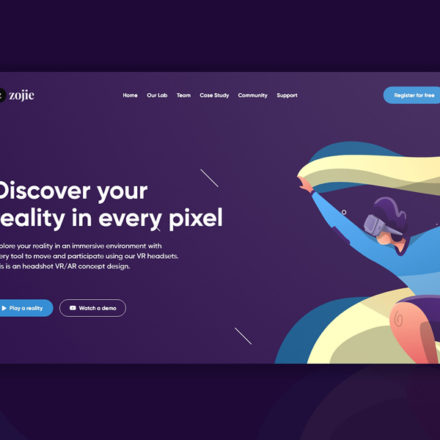This is an image captured from a screen, either of a cell phone or a computer. The top and bottom sections of the screen are bordered by rectangular bands of a deep bluish-purple color that is nearly black, with subtle hues of blue and purple visible.

Dominating the middle section of the image is a vibrant purple background, featuring the word "ZOJIC" in bold white print at the top. Beneath this header, there is a navigation bar displaying links labeled: "Home," "Our Lab," "Terms," "Case Study," "Community," and "Support." In the upper right corner, there is a prominent "Register for Free" button.

Centrally positioned on the purple background, the text "Discover your reality in every pixel" draws immediate attention. Below this tagline, a detailed graphic illustration shows a person with arms outstretched, wearing a cape-like garment and goggles. Small dashes, possibly representing raindrops, are scattered around the figure, adding a dynamic element to the scene.

Finally, at the bottom area of the screen, the text "Play a Reality" is displayed in blue, alongside another option, "Watch a Demo," which is set within the purple rectangle.